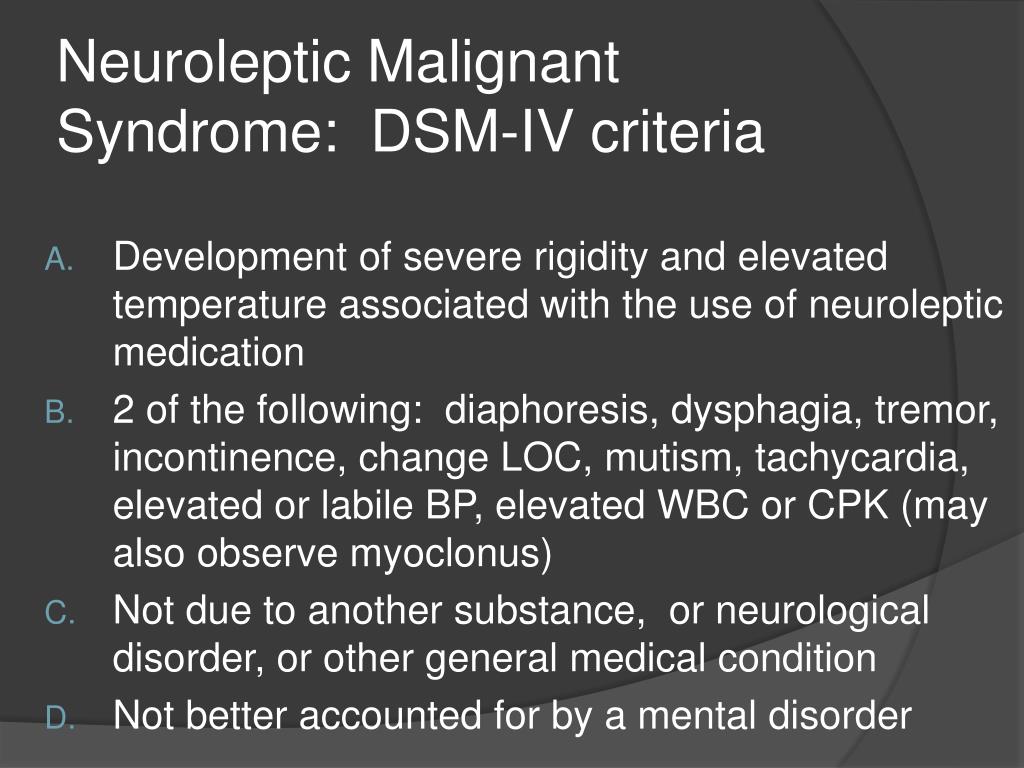The image displays text detailing the DSM-IV criteria for Neuroleptic Malignant Syndrome (NMS). The text is divided into several subsections:

- **Section A** specifies the development of severe rigidity and elevated temperature in connection with the use of neuroleptic medication.
  
- **Section B** lists additional symptoms for diagnosis, requiring at least two of the following: diaphoresis, dysphagia, tremor, incontinence, altered level of consciousness (LOC), mutism, tachycardia, labile blood pressure, elevated white blood cell count (WBC), or creatine phosphokinase (CPK). The observation of myokines is often noted as well.
  
- **Section C** clarifies that the symptoms must not be due to another substance, neurological disorder, or general medical condition.
  
- **Section D** states that the condition cannot be better explained by a mental disorder.

The text is in white and contrasts sharply against a gray background, making it stand out. The letters A, B, C, and D are highlighted in a darker green and blue gradient, providing a visual distinction for each section.